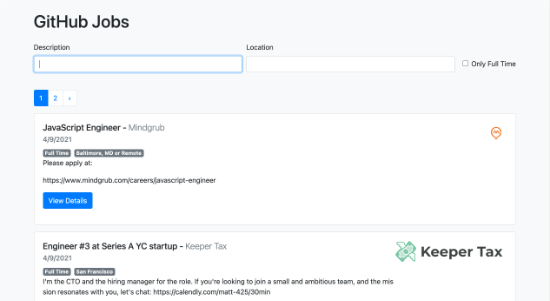The image depicts an interface of a GitHub Jobs web page. At the top, the "GitHub Jobs" header is displayed prominently against a white background. Directly below, there are two input boxes: one for a job description, which is currently empty, and another for a location, aligned horizontally. Additionally, there is a small checkbox labeled "Full Time," which is not selected.

Beneath these elements, pagination numbers “1” and “2” are shown, with number “1” highlighted in blue, indicating the current page. The first listed job is titled "JavaScript Engineer - Minegrub" and is dated April 9, 2021. This listing specifies that it is a full-time position located in Baltimore, Maryland. The complete location details are partially obscured. Instructions to apply are provided, directing users to the website minegrub.com/careers/javascript-engineer. A "View Details" button in bright blue is situated to the right of this listing.

The second job listing is for "Engineer #3 at Series A YC Startup - Keeper Tax," also dated April 9, 2021. It describes a full-time position in San Francisco. The post includes a message from the CTO and hiring manager, inviting candidates who resonate with the company’s mission to apply via a provided Calendly link: calendly.com/matt-425/30minute. To the right of this entry is the Keeper Tax logo, which features a green money icon.